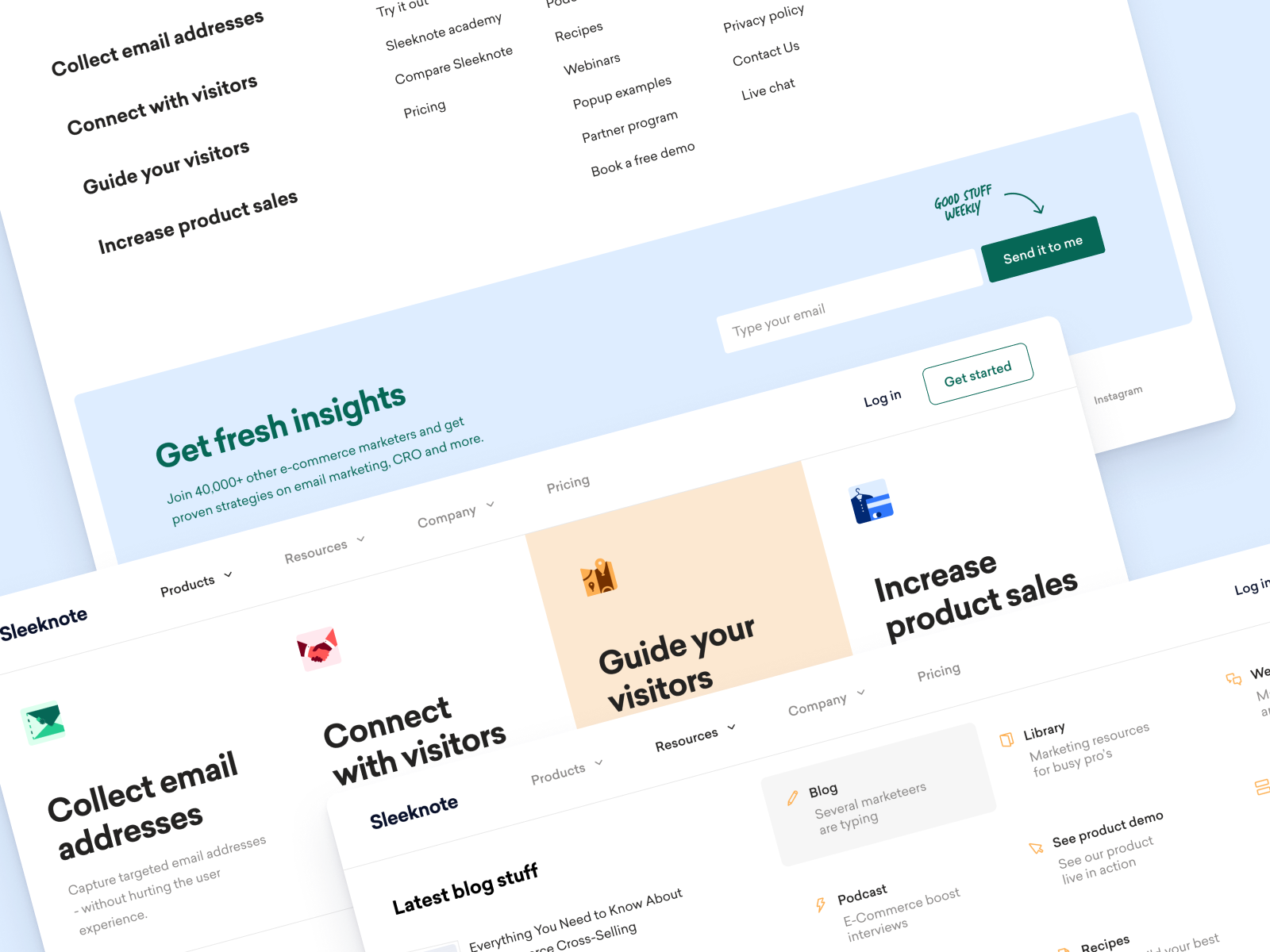In the screenshot, a computer or laptop display showcases an advertisement for “Sleek Notes,” highlighting an infographic related to the project. The image is set in landscape mode with a predominantly blue background. The infographic features a stack of white notes, each adorned with colorful accents, detailing the various features and benefits of Sleek Notes. 

The primary notes emphasize the capabilities of Sleek Notes, such as:
- Collecting email addresses
- Connecting with visitors
- Guiding visitors
- Increasing product sales
- Providing fresh insights to over 40,000 e-commerce marketers
- Offering proven strategies on email marketing and Conversion Rate Optimization (CRO)

Beneath these feature descriptions, there's an input field where users can type in their email addresses to receive more information and updates.

Additional notes on the infographic include options like pop-up examples, partner programs, pricing details, comparisons with other services, and access to the Sleek Note Academy and training materials. The notes are arranged in a diagonal layout, with each section expanding into drop-down menus for further guidance on how to enhance website visitor engagement and boost product sales.